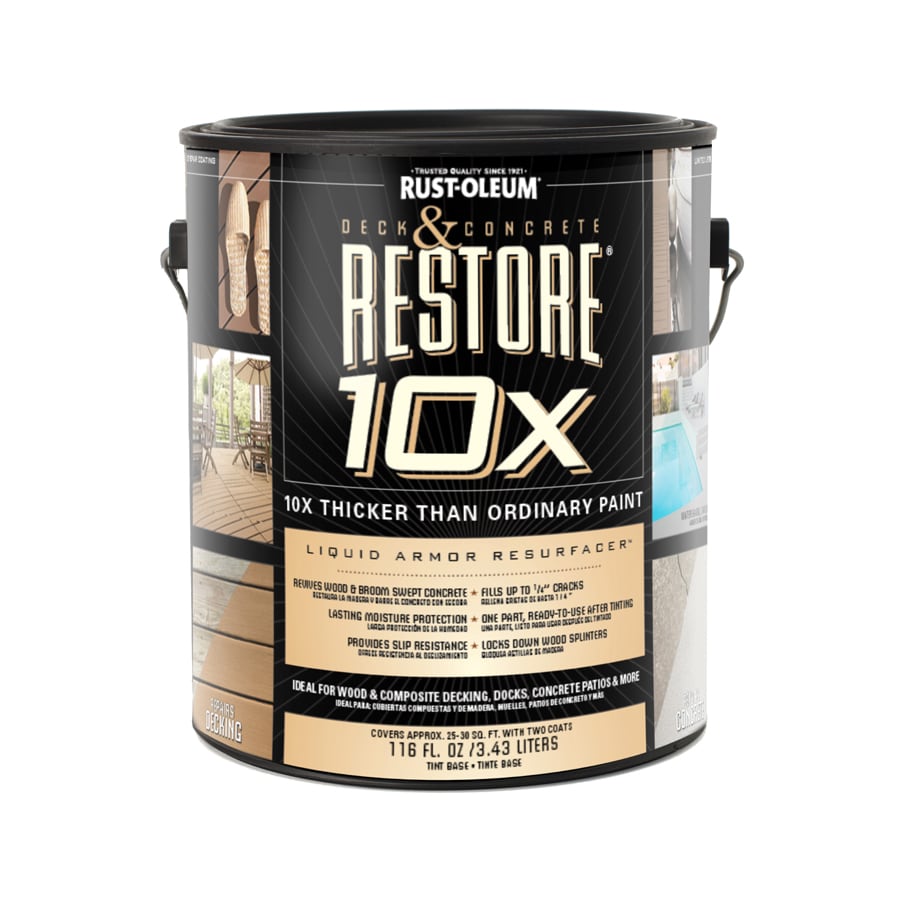This high-resolution stock photograph showcases a Rustoleum paint can against a seamless white background. The can's prominent black lid and label set a striking contrast, making the details easily legible. Dominating the upper section of the label, "Rustoleum" is emblazoned in bold white letters against the black backdrop. The central focus of the label reads "Deck and Concrete Restore 10X," emphasized in a robust font, highlighting its key feature of being "10 times thicker than ordinary paint." Below this, the label specifies "Liquid Armor Resurfacer," and lists its ideal uses for wood and composite decking, docks, concrete patios, and more. The label also includes illustrative before-and-after images of wood surfaces, providing practical examples of its transformative power. This versatile product is contained in a 116 fluid ounce can, and additional, smaller text details complete the comprehensive description, underscoring its high-quality, multifaceted applications.